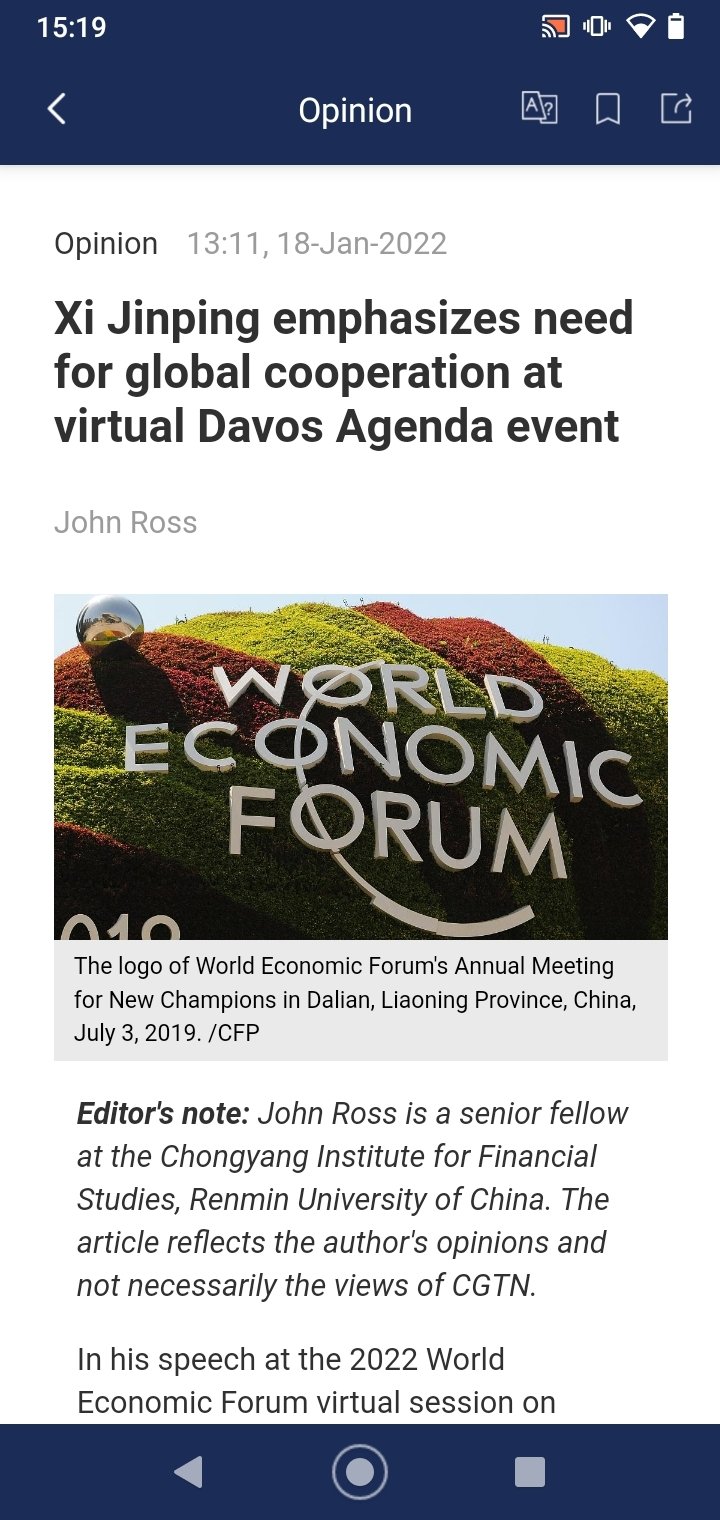A detailed screenshot from a smartphone is captured, featuring a navy blue border at the top. On the left of this border is the time displayed in a 24-hour format as 15:19. On the right side, several white icons indicate the battery life, Wi-Fi signal strength, and that the phone is on mute. Centrally positioned in this border is the word "Opinion" in white font, and to the left is a white arrow.

The main content of the screenshot showcases a webpage with a white background. At the top of this webpage, in gray font, the word "Opinion" is displayed alongside the date, "18 January 2022." Below this, a bold black headline reads, "Yao Ping emphasizes need for global cooperation at virtual Davos Agenda event." Beneath the headline, the journalist's name, John Ross, is written in gray font.

A photo is included in the article, featuring the words "World Economic Forum" in silver-gray font against a backdrop resembling hills. Beneath this image, the text reads: "The logo of World Economic Forum's annual meeting for new champions in Dalian, Liaoning province, China. July 3rd, 2019."

Further down, on the white background, an editor’s note states, "John Ross is a senior fellow at the Chongyang Institute for Financial Studies, Renmin University of China." The note also clarifies that "The article represents the author's opinion and not necessarily the views of CGTN."

The screenshot cuts off with the initial sentence of the article visible: "In his speech at the 2022 World Economic Forum virtual session on..."

The bottom part of the screenshot displays a navy blue footer. Within this footer, a gray circle is situated in the center, flanked by a gray triangle pointing left and a gray square on the right.